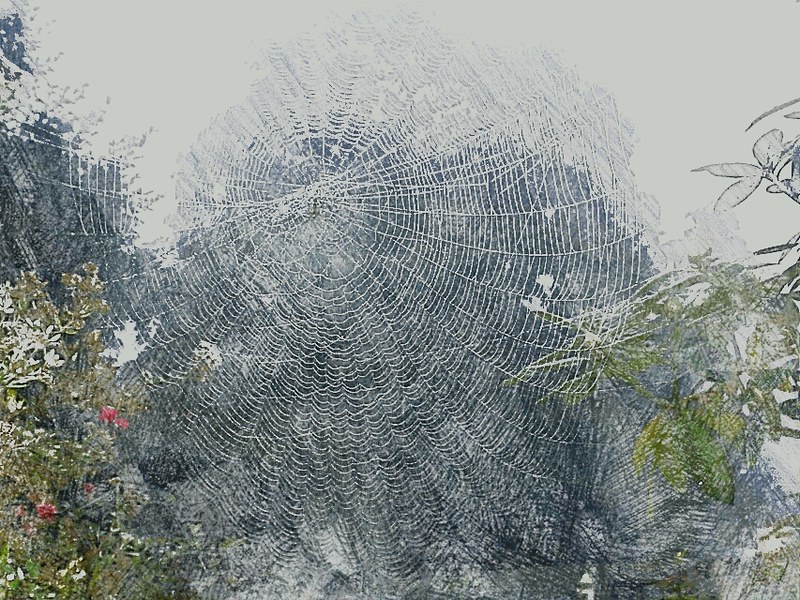This outdoor photograph prominently features a large spider web occupying most of the image, especially the center-left area from top to bottom. The web appears to be intricately woven between two trees, as evidenced by the leaves visible in the bottom right and bottom left corners. The tree on the right appears slightly higher than the one on the left. The background looks dark behind the web, with a bright, possibly daytime sky above it, suggesting it was taken during the day. A textured filter seems to have been applied to the image, affecting the appearance of the entire scene. This texture is particularly noticeable on the leaves of the right tree, which turn white and exhibit a distinctive pattern closer to the top. The colors in the image include whites, blacks, greens, pinks, and reds, and the overall effect gives the impression of either a stylized photograph or a piece of artwork. The image could be seen as looking through a window at the outside, reinforcing the idea that it might be a painting or an artistic rendition of a natural scene.